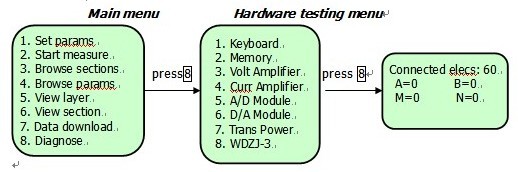The image is of a flowchart displayed on a white background, comprising three light green boxes with rounded corners and black text. At the topmost part of the image, the words "Main Menu" are prominently displayed. Below this header, the first light green box lists the following items in sequence: 1. Set Params, 2. Start Measure, 3. Browse Sections, 4. Browse Params, 5. View Layer, 6. View Section, 7. Data Download, 8. Diagnose. An arrow labeled "Press 8" points from this box to the second box.

The second green box is titled "Hardware Testing Menu" at the top. It contains the following items: 1. Keyboard, 2. Memory, 3. Volt Amplifier, 4. Curr Amplifier, 5. AD Module, 6. DA Module, 7. Trans Power, 8. WDZJ-3. Another arrow labeled "Press 8" directs to the final box.

The third and final light green box states "Connected to ELEC S: 60" at the top. Below this, two columns of parameters are listed: the first column reads A=0 and M=0, while the second column presents B=0 and N=0. Each of these green boxes is visually linked by arrows, forming a coherent flowchart that guides through various menu stages and settings.